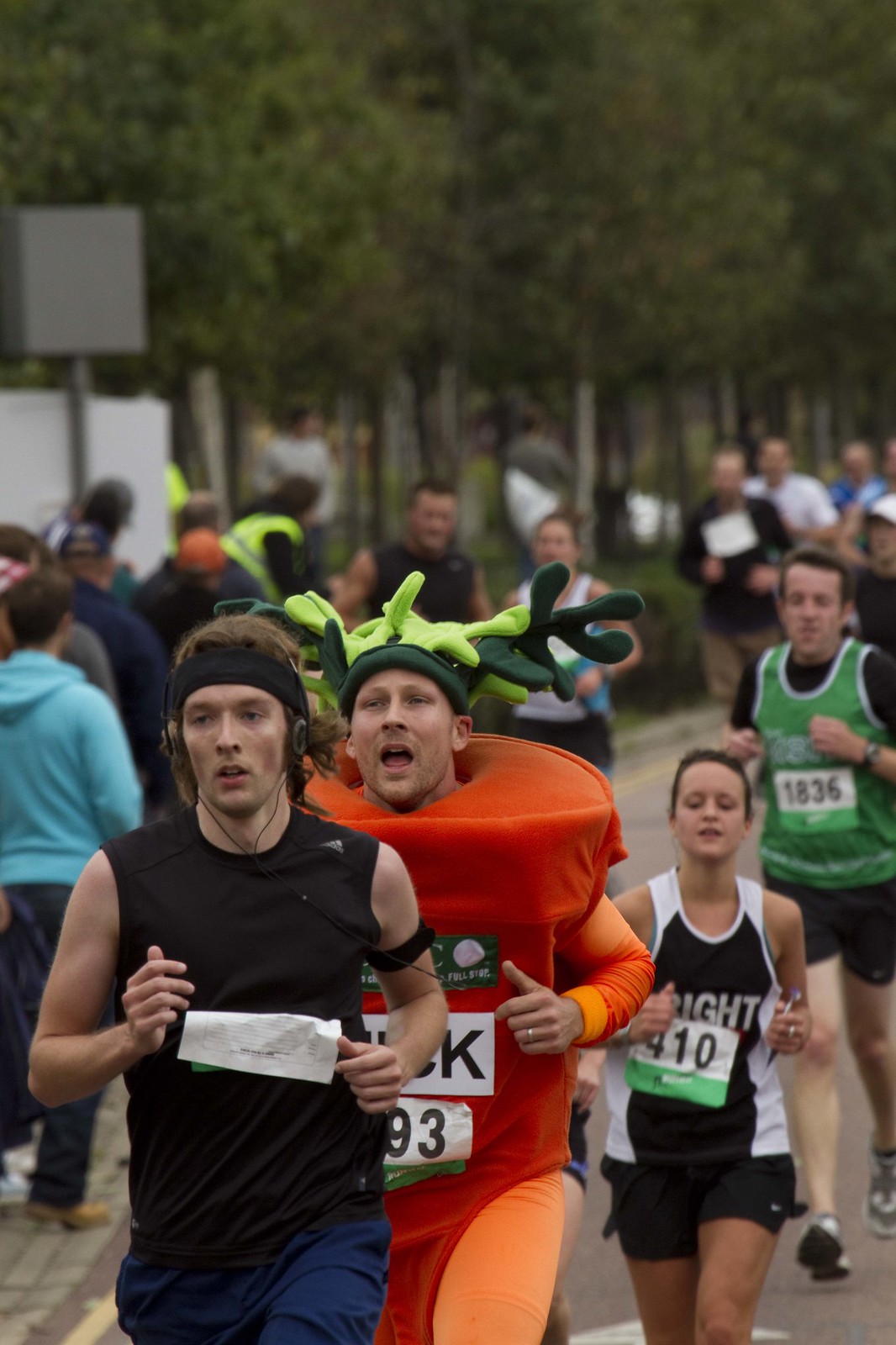This color photograph captures a bustling outdoor scene during a lively race event set against the backdrop of a park. In the foreground, a group of runners predominates the image. Leading the pack is a man in a black sleeveless shirt, blue shorts, and a black headband, listening to music through his headphones. His race number is partially folded and barely visible. Trailing closely behind him is a man in an eye-catching carrot costume, complete with an orange bodysuit and green leafy headpiece. Further back, a young woman wearing a green and white tank top with the number 410 prominently displayed jogs alongside a man in a light green shirt bearing the number 1836. Both are dressed in typical jogging attire.

Spectators line the sides of the street, their figures blurring into the background, capturing the energy and excitement of the race. The scene is framed by subtle details like trees with slender trunks and various signs to the left. The distant park adds a touch of greenery and openness, complementing the vibrant rush of participants in the center of the action.